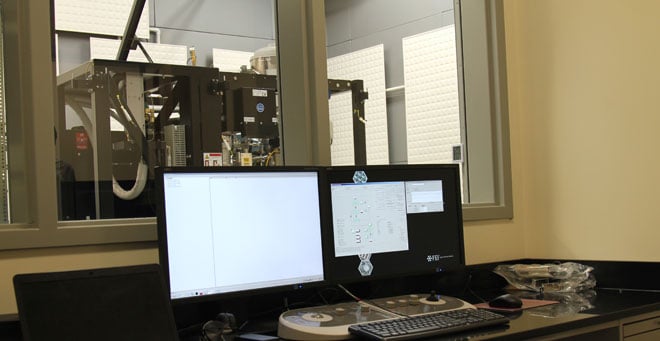The photograph captures the interior of an office, centered around a sleek, black desk setup. Prominently featured are two computer monitors; the left monitor displays a light-colored workspace that suggests it could be used for design purposes, while the right monitor shows two open boxes with flowcharts and hexagon shapes, indicative of a 3D printing interface. Positioned in front of the monitors is a black keyboard, and just above it, there is a joystick-like control panel. A black mouse rests on a beige mousepad to the right, next to which is a glass object that may or may not be an ashtray.

A large window, framed in gray, is situated behind the desk, offering a view into an adjacent room filled with mechanical or 3D printing equipment, including black boxes with visible motherboards and wires. The office walls are beige, and the overall setting is brightly lit. The workspace appears meticulously organized, suggesting a professional environment tailored for controlling or interacting with the machinery in the adjoining room.